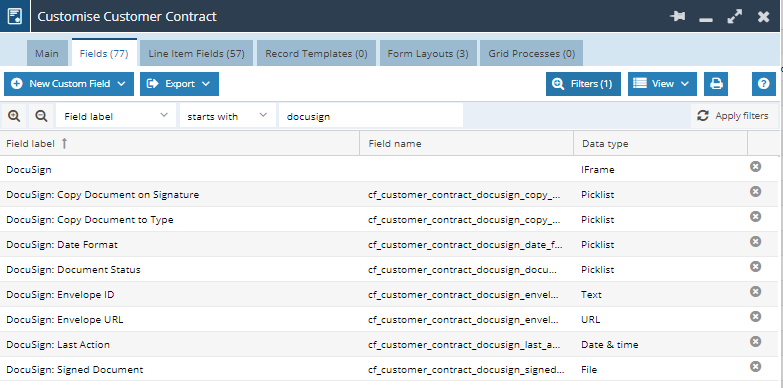This is a detailed left-to-right horizontal image of a computer screen interface. The background features a gradient that transitions from white at the bottom to gray and navy blue at the top. 

In the upper left corner, a white icon is visible against a teal blue background. Moving rightward, a navy blue banner stretches across the top, displaying the text "Customized Customer Contract" in white font. To the far upper right, icons for star, minimize, increase, and close (X) operations are present.

On the left side of the screen, text reads:
- "Main and Line of Fields (77)" – this section is highlighted.
- "Line Item Fields (57)"
- "Record Template (0)"
- "Form Layouts (3)"
- "Grid Processes (0)"

Below this text are buttons labeled "Add Custom Field," with an arrow pointing downward, and an "Export" button. As you move to the right, additional features include:
- Filters
- View options
- Print icons
- A Help button

The main body of the image contains a labeled chart, with columns titled "Field Label," "Field Name," and "Data Type." The initial entries under "Field Label" are "DocuSign" and "DocuSign - Copy Document with Signature." Each data entry can have a "Field Name" and a "Data Type," which may include options such as iframe, pick list, text, URL, date and time, or file. Each row in this section ends with a clickable grey circle containing an X.